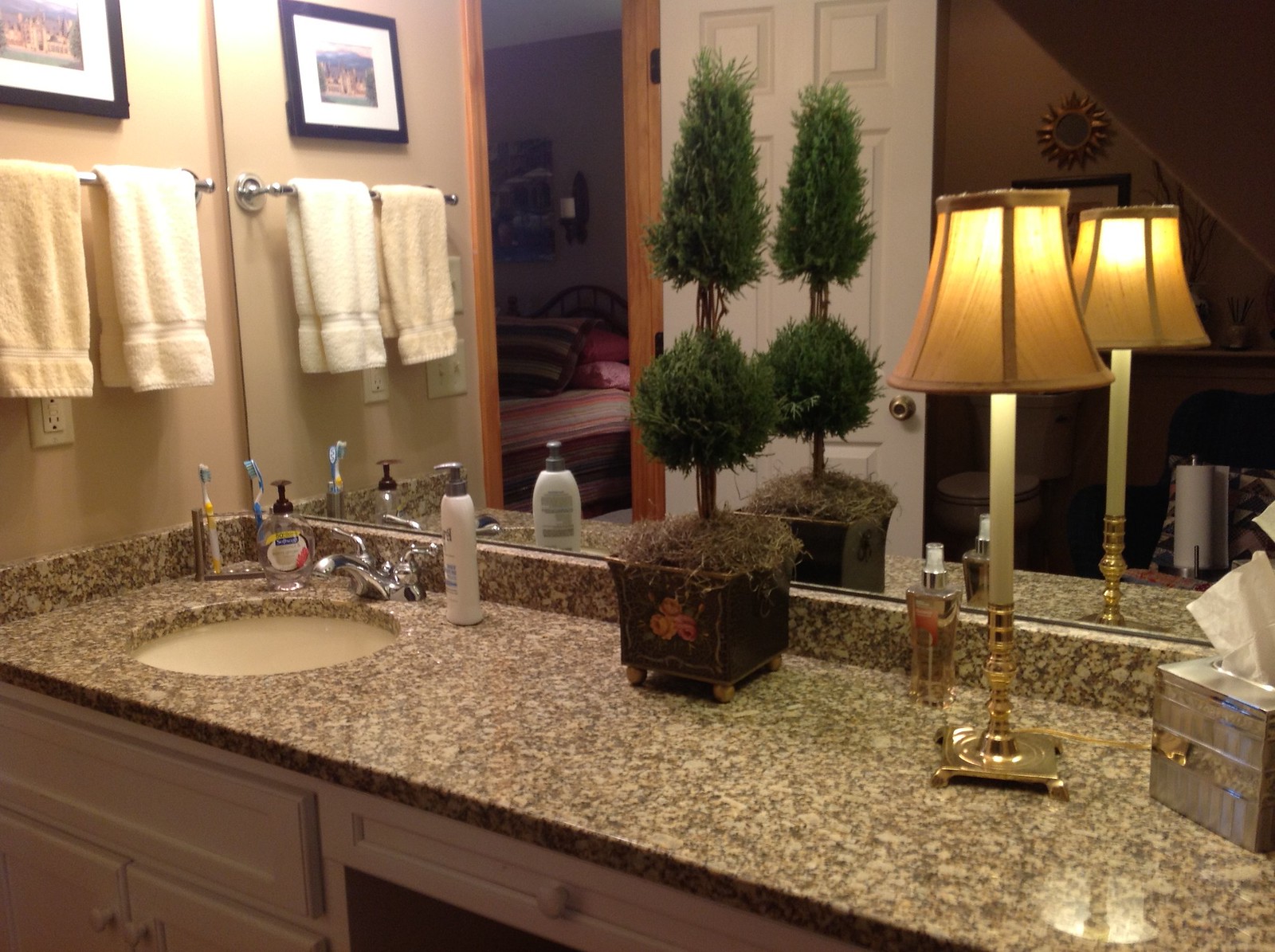The bathroom in the image appears to be part of a well-appointed home, exuding a sense of elegance and comfort. Central to the scene is a sleek sink set against a luxurious granite countertop. Atop the counter, there is a small, stylish lamp casting a warm glow across the space. Positioned near the lamp, a bottle of perfume adds a touch of sophistication. To the right of the lamp sits a neatly placed box of Kleenex, all contributing to a tidy and refined aesthetic.

Adding to the decorative elements, a small potted plant brings a hint of nature into the room. Adjacent to this greenery is the sink area, neatly organized with essentials such as lotion, hand soap, and two toothbrushes. To the left of the sink, mounted on the wall, is a towel rack holding two hand towels, further enhancing the room's functional appeal. Above the towels, a photo provides a personal touch.

A full mirror behind the sink area not only reflects the bathroom details but also offers a glimpse into the adjoining bedroom. In the mirror’s reflection, one can see the bathroom door and part of the bedroom, including a bed adorned with a maroon-colored bedspread. The bedroom walls, painted in a similar dark hue to the bathroom, contribute to a cohesive design theme. Additionally, a sconce with a candle above the bed is discernible, adding to the inviting ambiance of the living space.